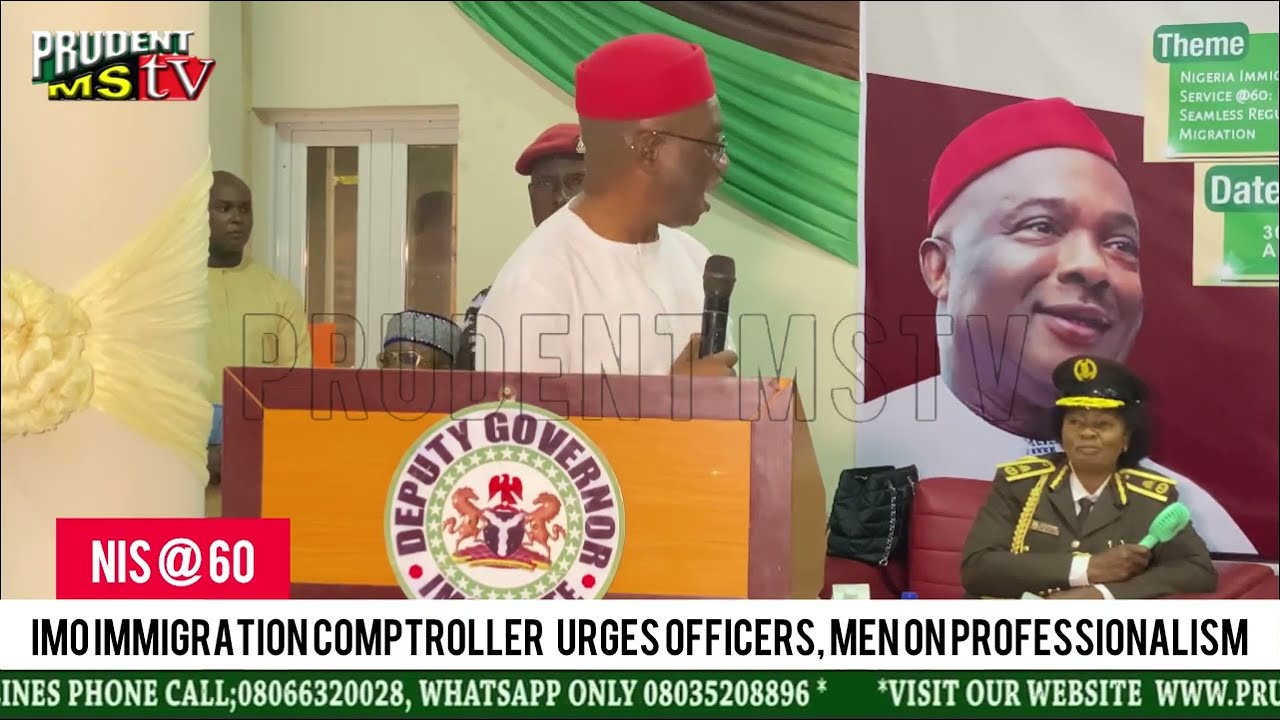This image is a screenshot from a television program, likely news coverage, featuring the Prudent MSTV logo in the top left corner. Central to the image is a black man standing in front of a podium, which bears a sticker reading "Deputy Governor." He is holding a microphone, dressed in a white t-shirt and a red hat, and is turning to look at a woman in a military uniform seated below a poster of a man also wearing a red hat. The woman’s uniform includes a hat with a gold leaf insignia and rank epaulettes on her shoulders. She is holding an indistinct green object that resembles a hairbrush. 

In the background, there are several other individuals, some standing and some barely visible behind a door. The upper part of the screen has additional graphics with text that reads "NIS at 60," and the main banner at the bottom states "IMO Immigration Comptroller urges officers, men on professionalism," despite some spacing issues making it difficult to read. There are further contact details partially visible at the bottom, including phone numbers and a truncated website URL. The scene appears to be indoors at a news conference.